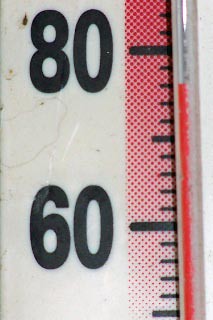The image captures the side of an analog thermometer against a white background. Dominating the view is the number "80" in bold black text, with the number "60" positioned approximately two inches below it. To the left of the number "80" is a small brown dot. To the right, the background features a decorative pattern of red and white boxes that gradually fade to white as they move downward.

From the top of the thermometer, there are two tiny black lines followed by a bolder black line, then four more tiny black lines, another medium-sized black line, four more tiny lines, another bold black line, and finally four more tiny lines leading to another medium-sized line at the bottom. To the right side of the thermometer, there is a section that fills with red fluid to indicate the temperature. In this image, the red fluid stops just two lines below the bold black line marking the number "80", suggesting a temperature slightly lower than 80 degrees.